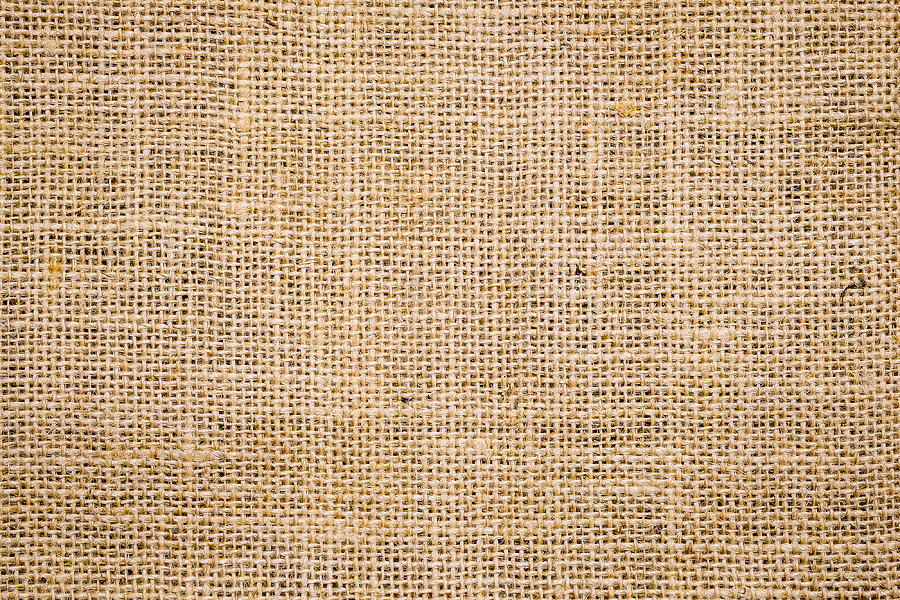This is a highly detailed, close-up photograph of a woven piece of fabric, resembling burlap or a similar rough-textured material. The image is slightly wider than it is tall, emphasizing a landscape orientation. The fabric, primarily light brown or tan, displays a tightly woven, grid-like pattern, with small square holes interspersed throughout. The texture suggests it is somewhat coarse, akin to burlap or the material used for potato sacks.

The fabric appears worn and stained, indicative of frequent use. Orange stains and random black and white fibers can be seen embedded within the weave, contributing to its aged and somewhat dirty appearance. Despite the signs of wear, the pattern remains symmetrical and consistent, with no visible cuts or tears.

The photograph is taken during the daytime, capturing the fabric in natural light, which highlights its details without any shadows. The image is entirely focused on the fabric, with no background elements visible, providing an intimate view of its texture and imperfections. The absence of edges or borders suggests the photo captures just a small portion of a much larger piece. 

In summary, this image presents a zoomed-in, detailed view of a woven fabric, its coarse texture, and visible signs of use, offering an intimate look at its intricate, grid-like pattern.